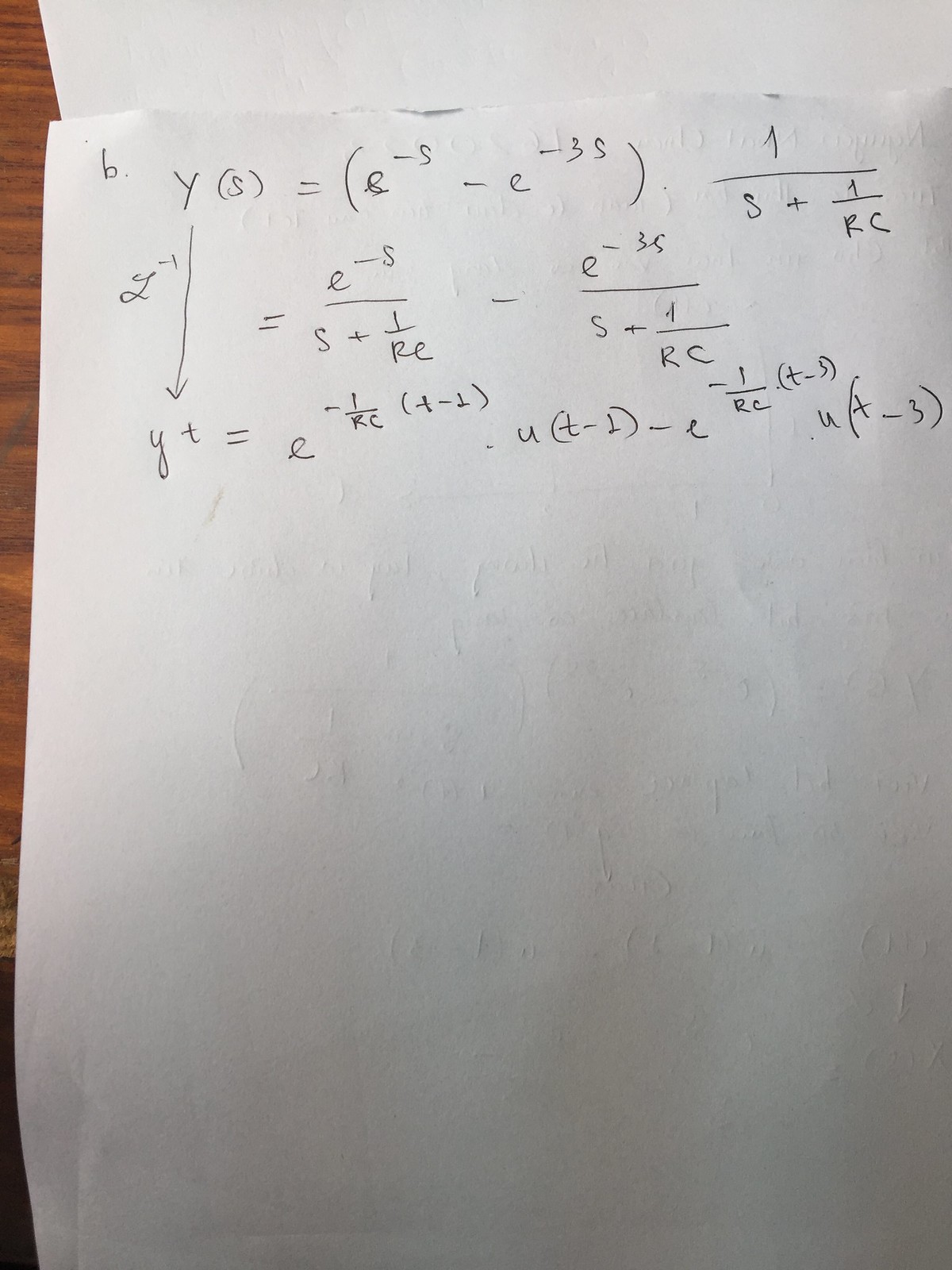A white sheet of paper lies on a rustic wooden surface, bearing the visible imprints of handwritten algebraic work on both sides. The front of the sheet prominently features a section labeled "b," indicating that the equations and derivations pertain to part 'b' of the problem set. Among the equations present, one stands out: \( y_s = [c^{-s} - e^{3s}] \). Below this initial equation, a step-by-step progression continues as the complex algebraic problem unfolds, showcasing various stages of the solution process meticulously written in pen. The faint imprints from the opposite side add an additional layer of texture, hinting at the thoroughness with which the problems have been tackled.